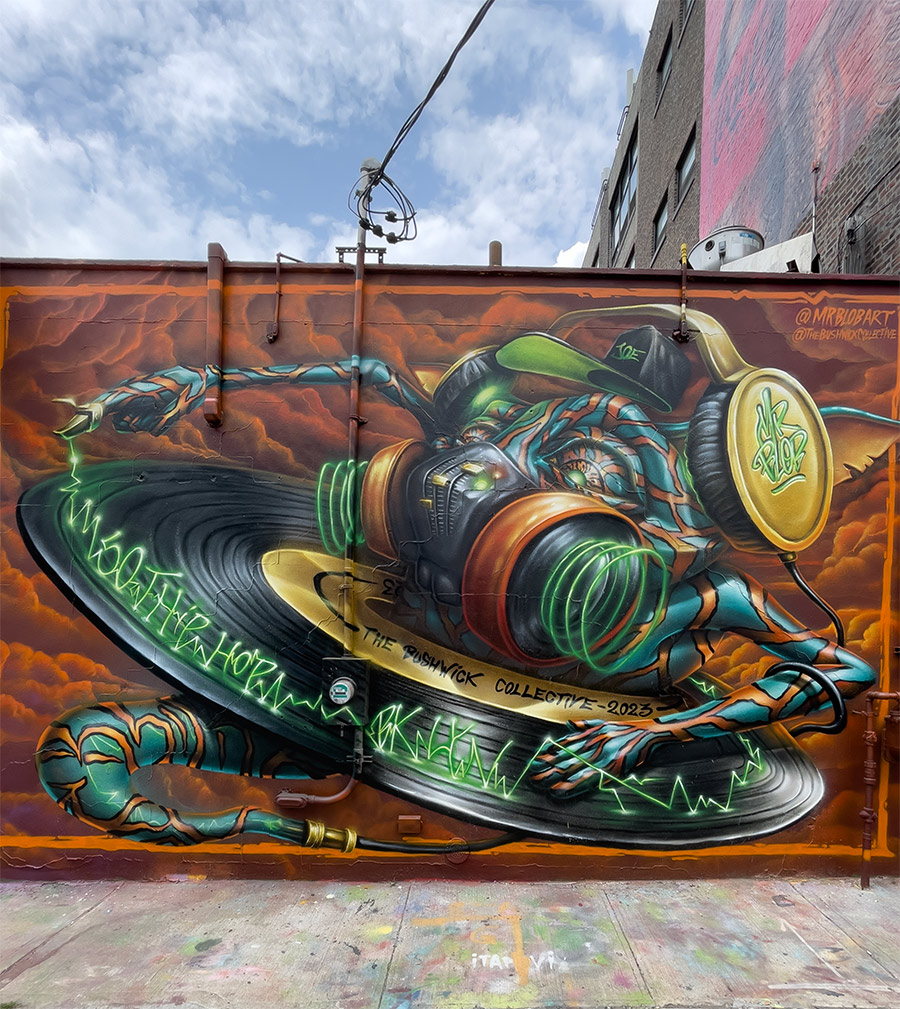The image is a detailed and vibrant digital photograph of a professionally done piece of sanctioned street art on Wall Street. The graffiti, painted on a low, flat stone wall, is highly polished and well-executed, deviating from the typical impromptu nature of most graffiti. 

The centerpiece of the artwork is an iguana-like creature, intriguingly positioned through the hole of a vinyl record. Surrounding the record's inner layer is black text that reads "The Posh Wick Collective 2023." The iguana, adorned with a face mask, adds a modern and edgy vibe to the illustration. Emerging from the iguana's finger is a neon, cursive inscription stating "M50 Dip Hop BKNYN," lending a dynamic and contemporary touch.

Incorporated into the artwork are a pipe and an electrical cable running vertically down the center, both seamlessly integrated into the painting, except for an unpainted meter on the pipe. The vibrant color palette includes shades of yellow, black, green, orange, gray, blue, red, and white, contrasting vividly against the backdrop of the stone wall.

The surrounding elements captured in the image include nearby buildings, the sidewalk beneath the wall, scattered clouds above, and several wires, adding context and depth to the urban setting of the scene.